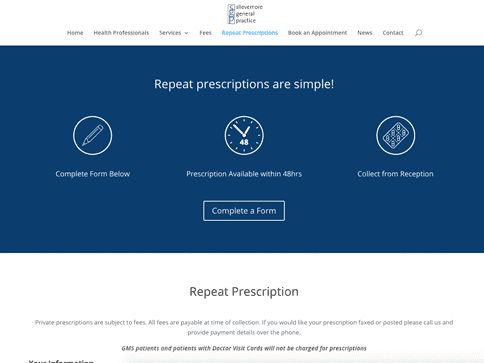The image is a screenshot of a prescription ordering website, which is somewhat difficult to decipher due to blurry text. The website appears to be named "Silver Something General Practice." 

At the top of the webpage, several tabs are partially visible, likely labeled as: Home, Health Professionals, Services, Fees, Repeat Prescriptions, Booking Appointment, and New Contact. A magnifying glass icon, presumably for search functionality, is also present.

Below the main navigation is a prominent navy blue box with white text that reads: "Repeat prescriptions are simple. Complete the form below. Prescription available within 48 hours, collect from reception." 

Central to the page is a clickable button labeled "Complete a form," inviting users to submit their prescription requests. Beneath this section, outside the navy box, is another heading labeled "Repeat Subscription," followed by smaller, barely legible instructions.